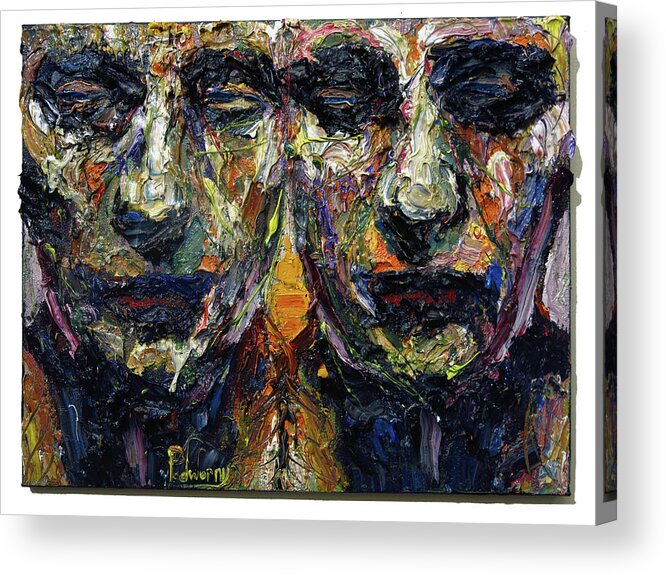The image is a framed painting with a white frame, featuring two closely resembling faces. These faces, which appear to be mirrored versions of each other, are depicted from just below the forehead to the upper chest region, with their heads and shoulders blending together in an abstract, almost fused composition. Both faces have their eyes closed, with black paint emphasizing the closed eyelids. The lips are vividly red, bordered with black and blue outlines. The artist employs thick pigments, daubed onto the canvas with a stick-like tool rather than a brush, creating a textured, three-dimensional surface. Dark shades such as black, dark purple, and blue accentuate the shadows around the eyes, mouth, and neck, while the nose, cheeks, and chin display brighter hues like white, green, yellow, orange, blue, pink, and purple. Under the chins of both figures, particularly beneath the one on the left, the darker paint creates an effect that could suggest a tie. The lower portion of the painting features the artist's signature, partially legible as "40." The word "power" is also visible, set against the white canvas background near the bottom. The bright yellow part between their faces adds a contrasting focal point to the overall composition.